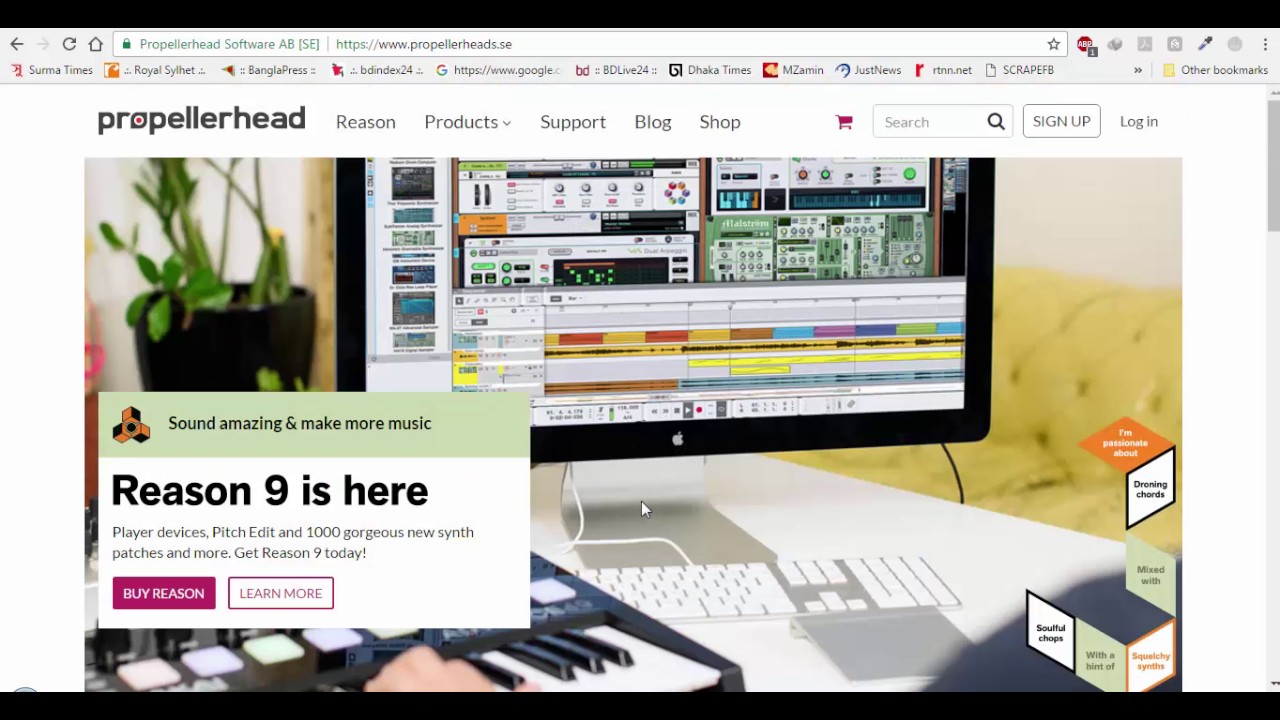**Caption:**

The Propellerhead Software webpage, specifically for their flagship product, Reason 9, is prominently displayed. At the top, the website navigation bar includes links to "Products," "Support," "Blog," and "Shop," along with icons for a shopping cart, search bar, sign-up bar, and login option. 

On the bottom left corner, a raised gray rectangle banner announces, "Sound Amazing and Make More Music. Reason 9 is here." Further details on the banner highlight new features such as Player Devices, Pitch Edit, and over a thousand new synth patches, urging visitors to "Get Reason 9 today" with options to either "Buy Reason" or "Learn More."

The central image features part of a musician’s workspace, including a keyboard partially obscured by a person's hand, an Apple Mac monitor, and another keyboard. In the background, there is a plant in a holder and a yellow leather couch situated on the opposite side of a modern, white table.